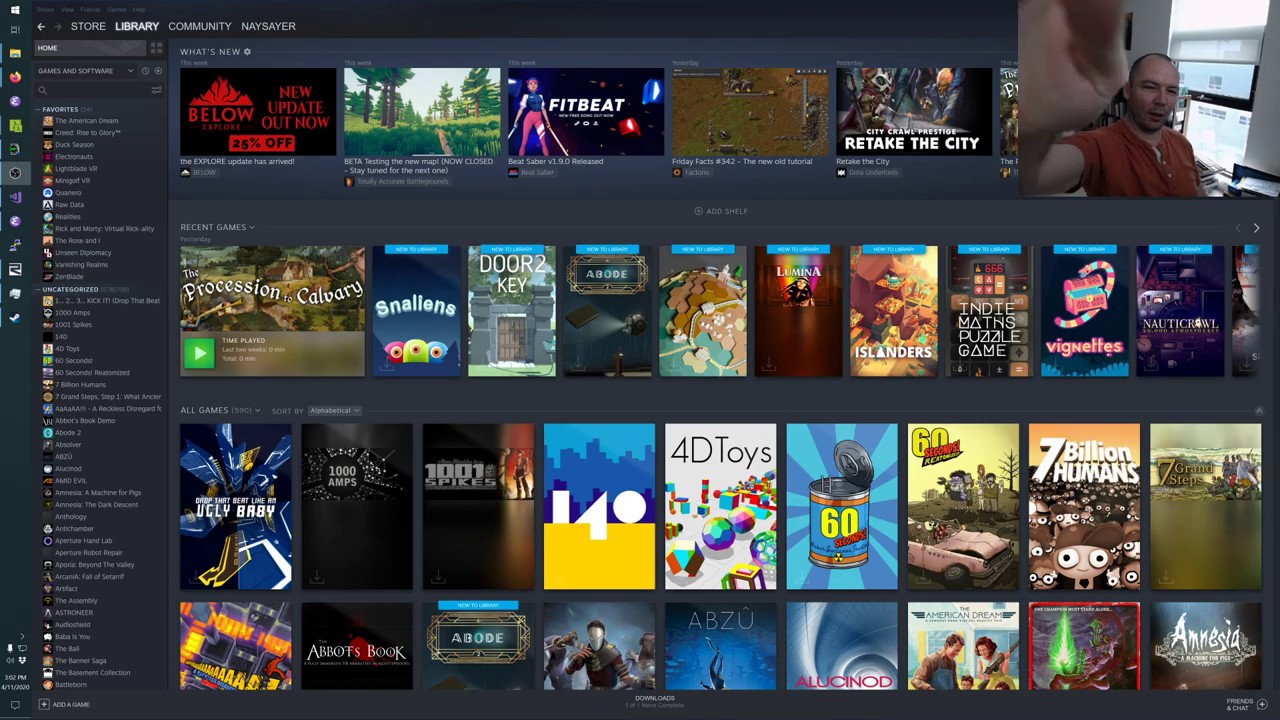The image displays a comprehensive website dedicated to a library encompassing various media such as books, audiobooks, and programs. At the top left corner, there are four categories labeled "Store," "Library," "Community," and "Saver," with the "Library" category highlighted in white, indicating the current section being viewed.

On the left side of the webpage, there's a sidebar menu, although the options are blurred and not legible. To the right of this menu is the main content area featuring several screenshots of available options. At the top of this section, two prominent options are displayed: "FitBeat," which appears to be related to exercise, and "Retake the City."

In the top right corner, there is a small window showing a person adjusting their camera, indicating a live user interacting with the app or website.

Below the main screenshots, there are three rows of additional options, each showcasing a diverse array of titles. The first row includes: 
- "The Procession Calvary"
- "Door to Key"
- "Islanders"
- "Vignettes"

The second row features: 
- "Ugly Baby"
- "1001 Spikes"
- "140"
- "40 Toys"
- A can labeled with "60"
- "7 Billion Humans"

The third row presents:
- "Epic Book"
- "Abode"
- "Abzu"

In the bottom right corner of the screen is the option labeled "Amnesia." Each row and option hints at a wide variety of content available within this digital library.